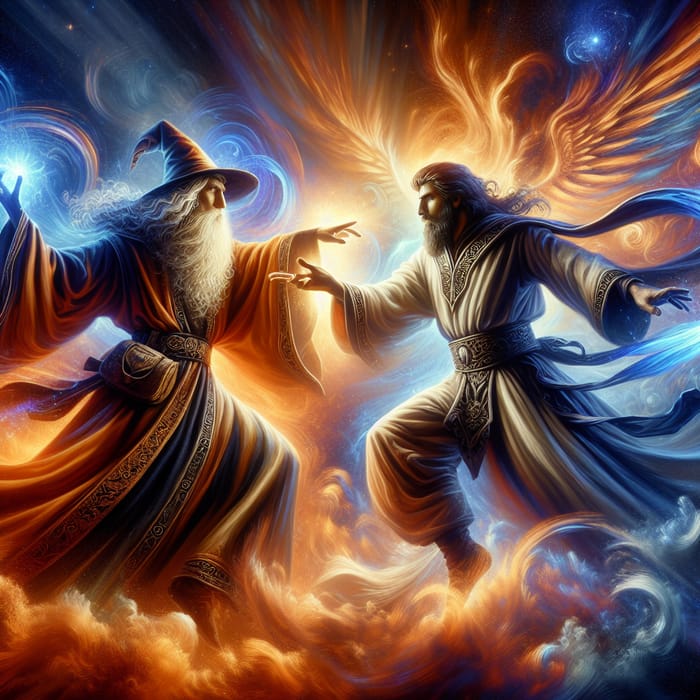The image is a detailed and highly colorful drawing of two wizards facing each other, seemingly ready for battle. On the left side stands an elderly wizard with long wavy white hair and a very long white beard. He is wearing an orange wizard's hat with a round brim, an elaborate orange and blue cloak, and a brown fanny pack attached to a belt around his waist. His left hand is casting a blue light that emanates dramatically from his hand. The wizard on the right has wavy brown hair and a shorter gray beard, and he is dressed in a silver robe with a darker silver belt. The background is filled with abstract swirls of bright oranges, blues, and clouds, creating a vivid scene that emphasizes the intensity of their confrontation. The overall artistic style is animated and striking, with a series of colored streaks and smoke lending a dynamic atmosphere to the scene.